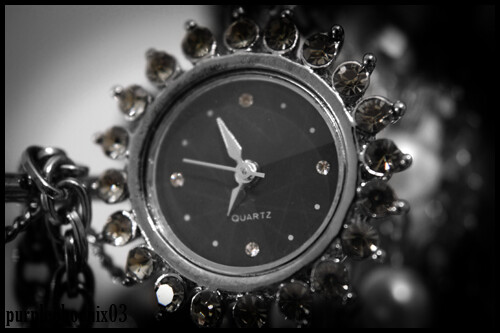This detailed indoor black-and-white photograph captures a close-up view of an exquisite circular watch, possibly a brooch-type timepiece, without a visible wristband. The watch face is entirely black, adorned with minimalistic hour markers where small dots denote the hours, and the positions of 12, 3, 6, and 9 are highlighted with larger, prominent diamonds. The watch indicates the time as 6:55, with the second hand positioned just above the nine o'clock mark, all hands rendered in a sleek, metallic silver color. The periphery of the watch face features a collection of gemstones set in silver, adding to its luxurious appearance. Clear, capitalized text reading "QUARTZ" is displayed just above the six o'clock position. The background transitions from a lighter hue on the left to a darker shade on the right, providing contrast to the focal watch. A chain is slightly visible in the lower left corner, hinting at the watch’s potential dual function as a brooch. The framing blurs out the background completely, ensuring the watch remains the central focus of this elegant and detailed depiction.